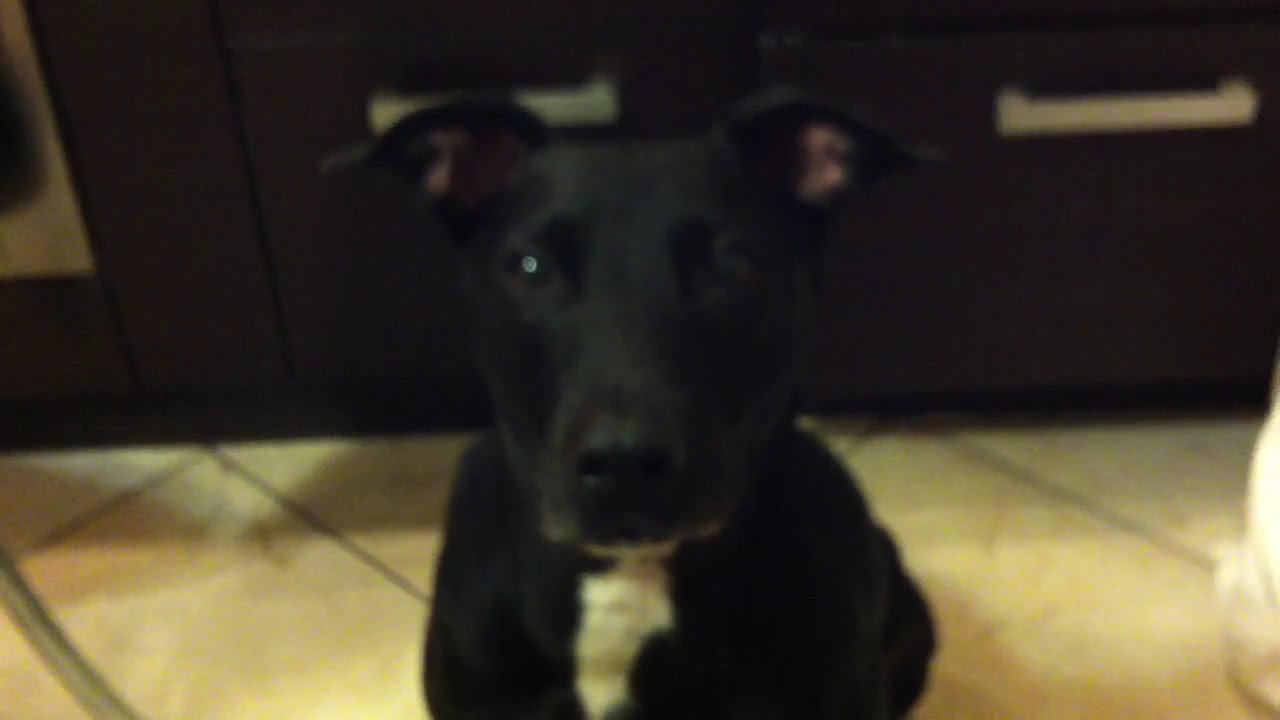The image captures an adorable, yet out-of-focus photograph of a black puppy dog sitting in the center, looking straight into the camera. The dog has a white patch under its chin running down its chest, and pointy, slightly floppy ears with pink insides. Its mouth is closed, and the puppy's expression is one of curiosity, staring intently into the lens. In the background, dark brown kitchen cabinets with white or silver handles are visible, suggesting the photo was taken in a kitchen. The flooring appears to be a cream-colored or light linoleum with a square pattern. There's a vague, white shape in the bottom right corner that is difficult to identify due to the image's blurriness. Additionally, another indistinct white-colored shape, possibly another animal, is on the left side of the frame, adding to the overall mysterious and domestic atmosphere of the photograph.